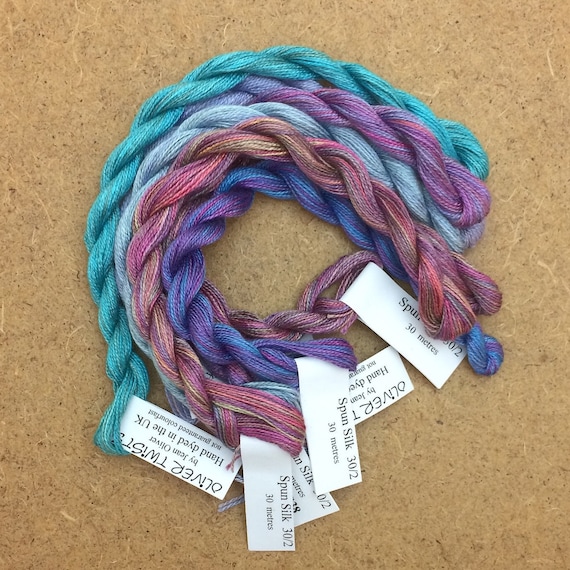The image displays a collection of hand-dyed, braided silk threads arranged on a cork-like background, which is a tan or brown color. Each silk braid features multiple intertwined colored strands, including vibrant shades of aquamarine, turquoise, blue, green, pink, mauve, burgundy, teal, and purple. The silk threads are meticulously crafted by Jean Oliver in the UK, and each thread is tagged with small white labels that read "Oliver Twists, by Jean Oliver, Handmade" on one side and "Spun Silk, 30/2, 30 meters" on the other. The braids are coiled into a C-shape, highlighting the range of their vivid colors and making them appear almost like artisanal, open-ended bracelets.